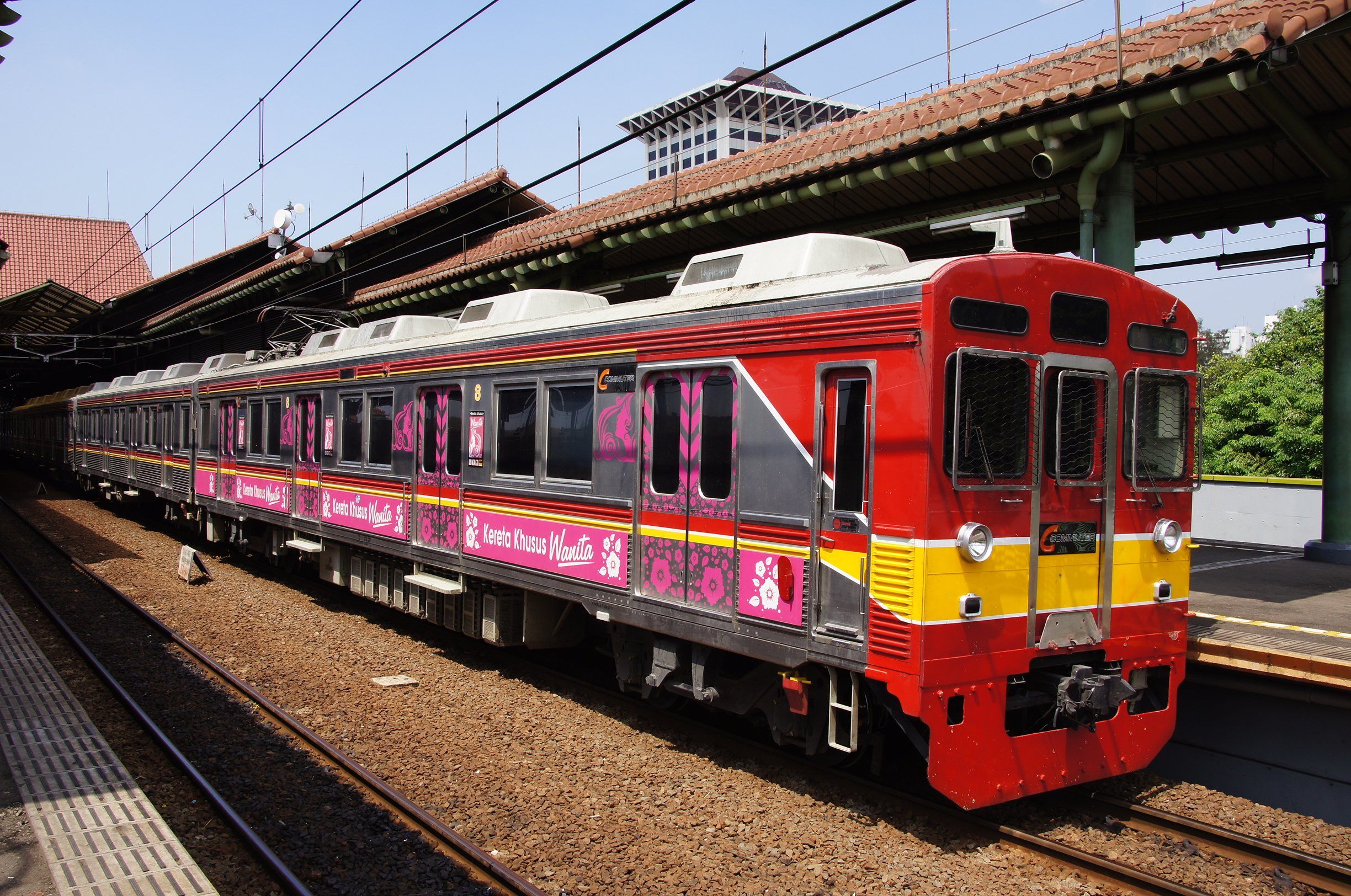The photograph, taken outdoors during the daytime, captures a stationary train at a train station. Overhead, a clear blue sky adds a sense of open space, while the outlines of buildings loom just above the station's red or brownish roof, providing an urban backdrop. High above the train tracks, cables thread through the scene, hinting at the electrical infrastructure.

The train platform itself has a clean, gray floor. The train rests on brown or copper tracks, with soil or wood chips surrounding them, adding a natural touch to the industrial setting. The train is primarily red, accented by a horizontal yellow stripe that runs through its center. On its side, pink advertisement signs and some white text, which is difficult to decipher, add splashes of color and commercial elements. The train's design is dominated by its large, square shape and a white roof, giving it a robust and modern appearance. Additionally, some faint hints of shrubbery can be seen on the right side of the photo, contributing to the overall detailed composition.